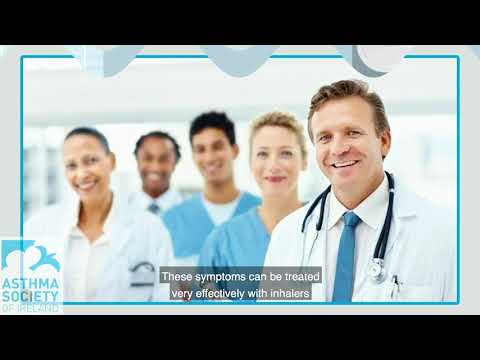This image is an advertisement for the Asthma Society of Ireland prominently featuring five medical professionals. On the far left, a woman with a short black buzz cut and all-of complexion stands wearing a white doctor's jacket and undershirt. She has a device in her right pocket. Behind her is an African American man with black hair, smiling, who is slightly blurred and dressed in a white shirt. Next to him, also somewhat blurred, is another man with a short black haircut and an all-of complexion, wearing a light blue shirt over a white undershirt. There’s a blonde-haired woman with reddish-pink lips and a blue nurse's uniform, clearly in focus, who is also smiling. The man in the foreground on the far right has brown hair and a mustache, smiling warmly as well. He wears a white lab coat over a white shirt and blue tie, and has a black and silver stethoscope around his neck. Visible on his lab coat is a pen in his pocket. In the bottom left corner of the image, there’s a logo for the Asthma Society of Ireland. A YouTube-style text overlay at the bottom of the image reads: "These symptoms can be treated very effectively with inhalers."